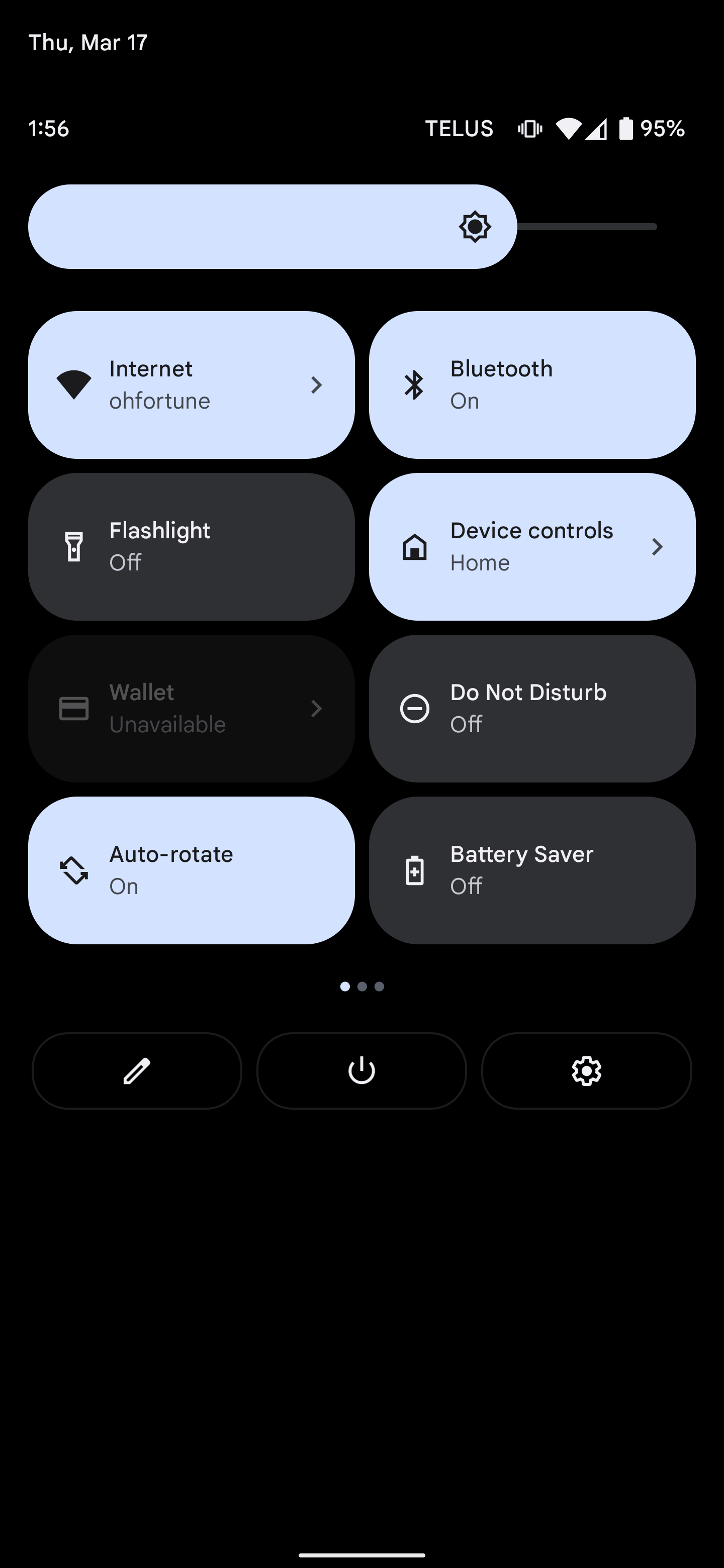Here is a detailed and cleaned-up caption for the image:

---

The screenshot displays the quick settings menu on an Android device, providing a snapshot of key device statuses and options as of Thursday, March 17, at 1:56 PM. At the top, the battery level is prominently shown at 95%. The quick settings tiles include:

- **Internet:** Connected to a Wi-Fi network named "Oh Fortune," indicated by a Wi-Fi symbol. 
- **Bluetooth:** Enabled, signified by a Bluetooth symbol.
- **Flashlight:** Disabled, with a corresponding flashlight symbol.
- **Device Controls:** Active for the current home setup, represented by a home icon.
- **Wallet:** Marked as unavailable, noted by a grayed-out wallet symbol.
- **Do Not Disturb:** Disabled, alongside a "Do Not Disturb" symbol.
- **Auto Rotate:** Enabled, depicted by an auto-rotate symbol.
- **Battery Saver:** Disabled, indicated by a battery saver symbol.

At the bottom navigation bar, there are three icons:
 
- **Edit (Pencil Icon):** For customizing quick settings.
- **Power Button Icon:** For power options.
- **Gear Icon:** For accessing device settings.

The layout is designed for swift and convenient access to frequently used settings, allowing users to enable or disable features quickly and efficiently.

---